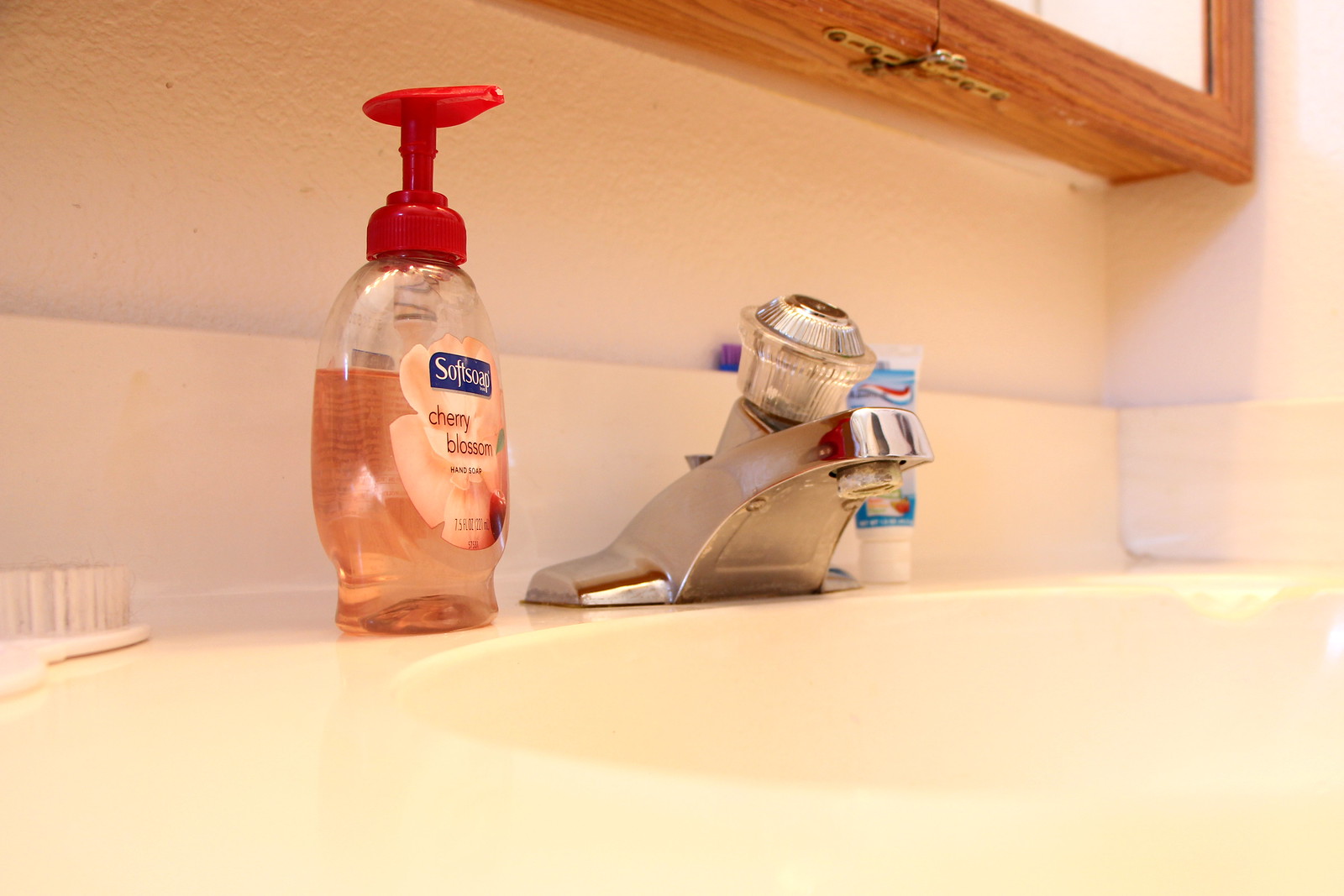This image showcases a pristine bathroom sink, centered around a sparkling white porcelain basin. The modern sink features a gleaming silver faucet with a clear, circular top. To the left of the faucet, there is a small, white brush positioned neatly. Adjacent to the brush, a soap dispenser stands prominently, labeled "Softsoap" in blue and white text with a cherry blossom design. The dispenser, which is approximately 75% full, sports a red plastic top, hinting at a fresh and intense floral fragrance. On the right side of the sink, partially obscured by the faucet, sits a miniature toothpaste dispenser, though its specific brand and details remain hidden. Above the sink hangs a modest wooden-framed mirror, completing the bathroom setup. The overall aesthetic is clean and minimalistic, providing a sense of order and freshness often reminiscent of a well-kept retail environment like Target.